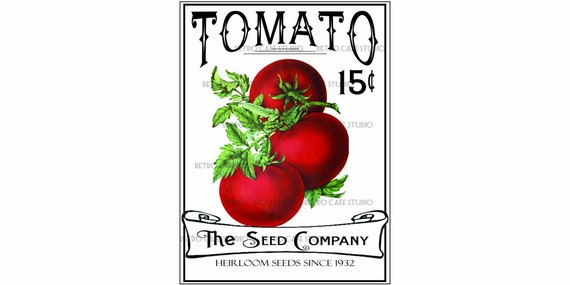This image showcases the front cover of a seed packet for tomato seeds, typically sold in grocery and hardware stores. The vertical rectangular artwork sits against a white backdrop framed by a thin black line. At the top, in bold black font, the word "Tomato" stretches across, followed by "15 cents" prominently displayed to the right. The central illustration features three red vine tomatoes, adorned with small green leaves, arranged vertically on the same vine. Below this vibrant illustration, a partially unfurled scroll depicts the words "The Seed Company" in distinct font, followed by "Heirloom Seeds Since 1932." The meticulously detailed design aims to attract those looking to cultivate tomatoes in the upcoming growing season, emphasizing the heritage and affordability of the seeds.